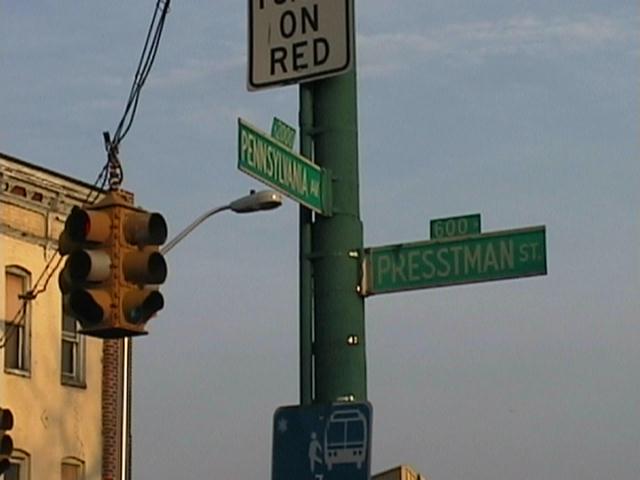In this outdoor scene, a prominent green metal pole stands at the center, adorned with various street signs. Set against a grayish-blue sky with wisps of thin white clouds, the pole features a green rectangular sign with white lettering on the right that reads "600 Pressman Street." On the left, a similar sign indicates "Pennsylvania Avenue." There's a partially visible white sign with a black outline at the top middle of the pole, where the word "red" is readable but the rest is cut off.

On the left side of the image, part of a beige stucco building with windows is visible. At the corner of this building, a traffic light hangs from a wire, although the actual lights are not discernible; only the housing for the three round lights is visible from two sides. Additionally, a metal lamp post is partially in view, extending down from the side of the building.